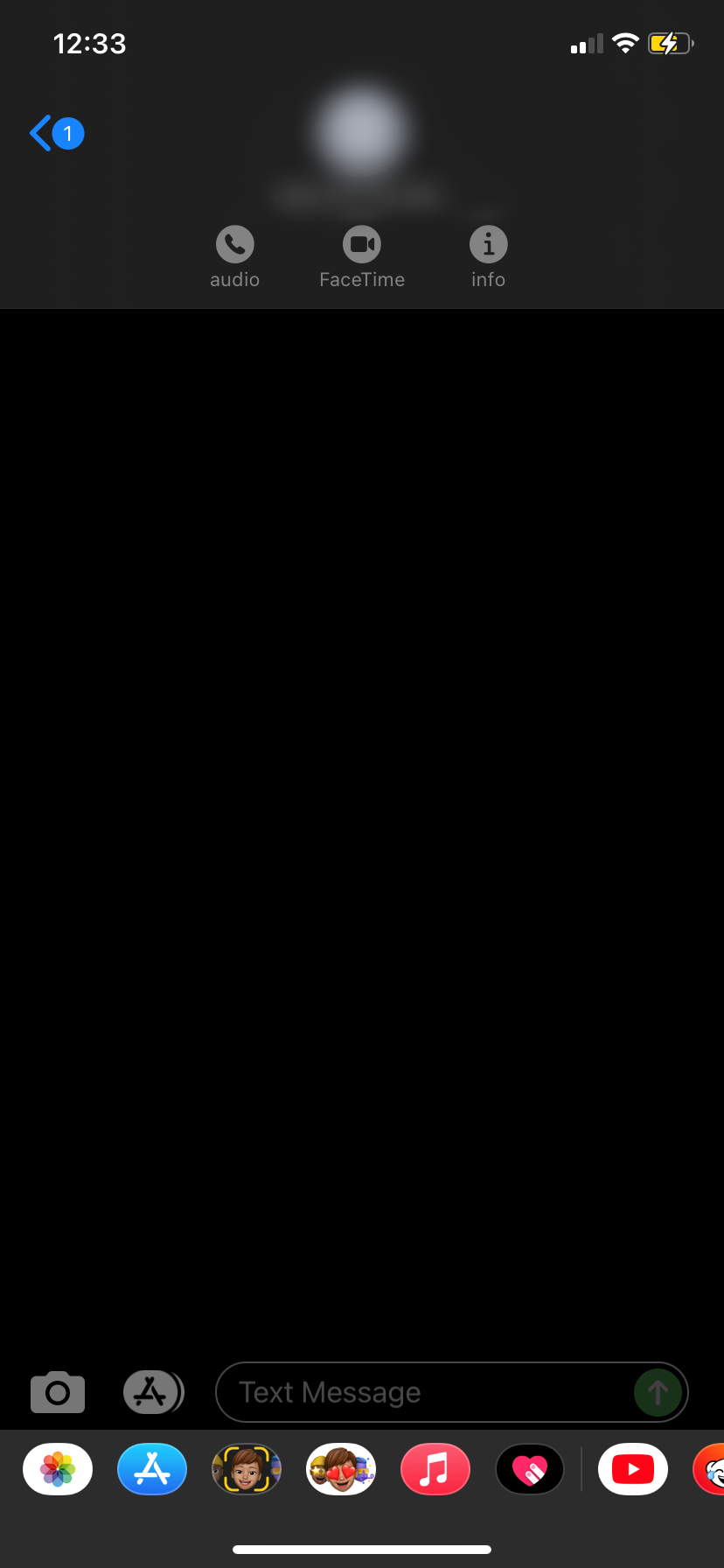The image depicts a blank text messaging screen on an Apple device in night mode. The screen shows a current time of 12:33 located at the top left corner. The signal strength appears to be two out of four bars on the right-hand side, alongside a fully strong Wi-Fi signal indicated by the maxed-out Wi-Fi icon. The battery icon shows the device is charging, with a lightning bolt symbol and a yellow fill.

Just below the time, a back arrow signifies there is one unread message or notification. The recipient's identity is blurred for privacy. Beneath the blurred name, there are icons for audio (represented by a phone icon), FaceTime (marked by a video camera icon), and information (indicated by an eye icon).

The main messaging area is entirely black, indicating night mode with no texts displayed. At the bottom of this section, icons for attaching a photo, the App Store, and typing a text message are visible. The camera icon, App Store (depicting pencils forming the letter 'A'), and a greyed-out green circle with an upward-facing white arrow for sending messages are included.

At the bottom of the screen are various app shortcuts. These include:
- Photos, depicted by a rainbow flower-like icon.
- The App Store, again symbolized by the letter 'A' formed by pencils.
- Two custom avatar icons for user-created emojis.
- Apple Music, shown as a pink capsule with music notes.
- Another app represented by a black icon with a pink bandaged heart.
- YouTube, indicated by a rounded rectangle with a right-facing arrowhead.
- A final icon, possibly representing Reddit, though not clearly identifiable.

In summary, the screen shows an active Apple messaging interface in night mode with no current messages displayed and several app integrations visible for quick access.